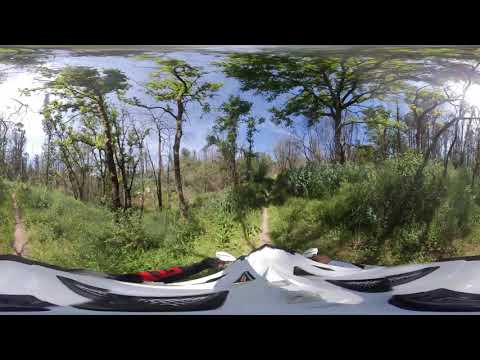This image, captured outdoors with a fisheye lens, presents a panoramic view of a serene forest scene. The photo has a wide-angle composition, framed by black borders on the top and bottom, where the curvature typically associated with fisheye lenses is not apparent. At the forefront, there is a subtle distortion suggesting a white object which could possibly be a drone hovering, faintly noticeable amidst the greenery.

The scene extends into a rough, untamed forest characterized by a moderate density of green trees with either black or brown trunks, interspersed with shrubs and abundant grassy vegetation underneath. Distinguished in the middle, a narrow, possibly sandy footpath meanders into the heart of the forest, directing the viewer's eye towards the horizon. Additional trails or dugouts appear scattered around, enhancing the rustic aesthetic.

The forest lacks a dense canopy, allowing light to filter through, and the day is bright and sunny as evidenced by the light blue sky adorned with a few fluffy white clouds. No human presence is visible, emphasizing the untouched, wilderness aspect of the environment. The image overall suggests a tranquil and natural setting, where the beauty of an unmanicured forest is prominently displayed.